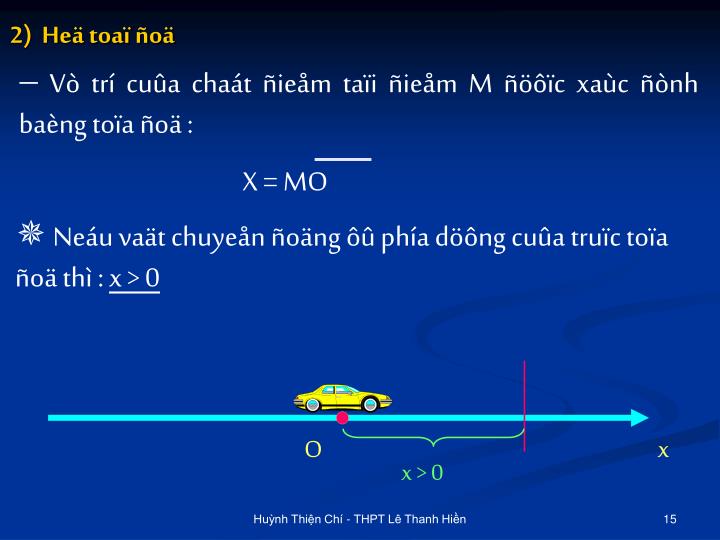The image is a digital presentation slide with a blue background that transitions to black near the top. At the top left, there's a yellow number "2" followed by non-English text featuring many diacritics, suggesting it could be in a Southeast Asian language. Below this, there's an equation "X = MO" with a line above it, followed by additional text that mentions "X > 0." The slide features a graphic of a small yellow car on a light blue arrow pointing to the right, with a red dot under the car and a red line some distance in front of it, connected by a bracket indicating the distance as "X > 0." In the bottom right corner, there's a light-colored "15" and some small white text that may be the presenter's name.